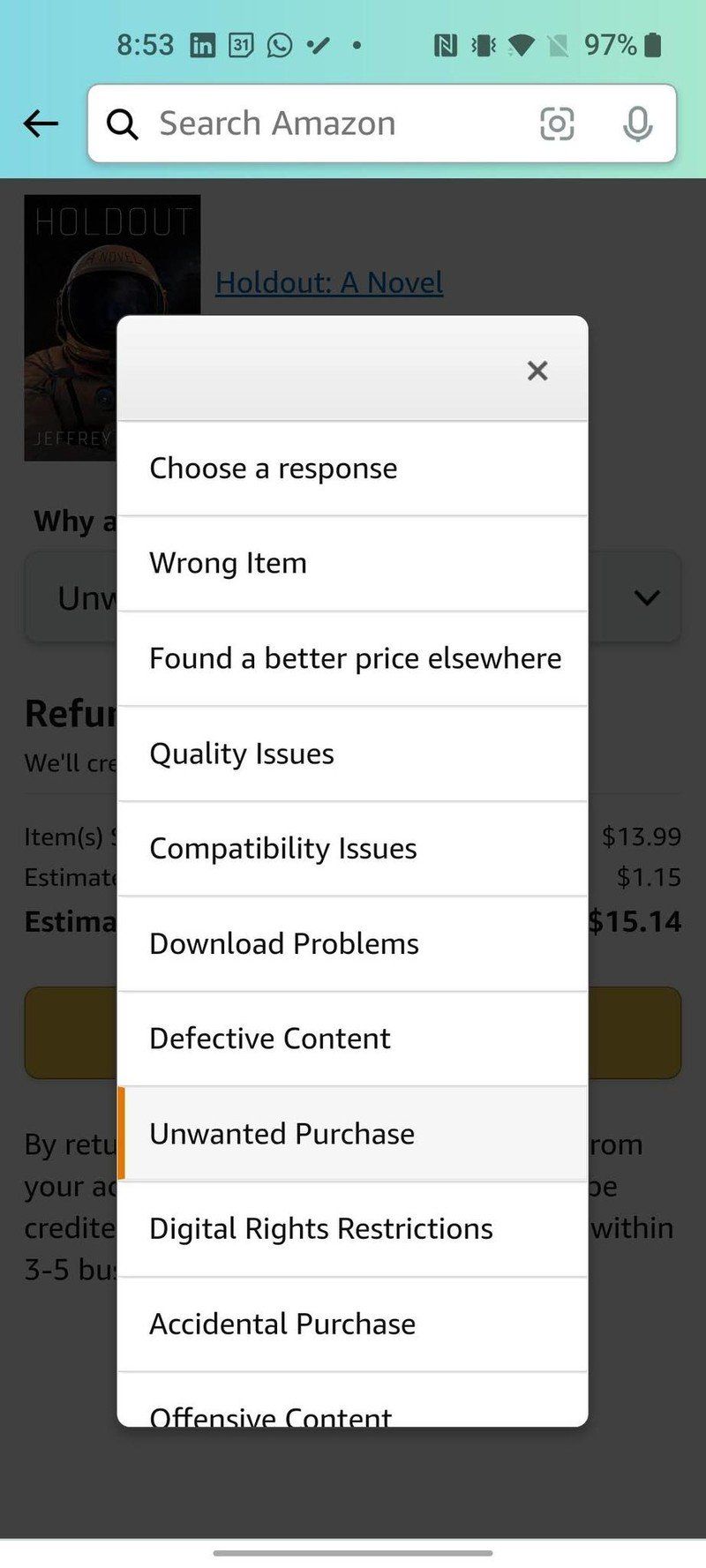Screenshot of a smartphone display at 8:53 AM with a 97% battery level. The screen features a prominent Amazon search bar at the top. Below the search bar, a large pop-up window titled "Choose Response" lists various options for addressing an issue with a purchase. The options include: Wrong Item, Found a Better Price Elsewhere, Quality Issues, Compatibility Issues, Download Problems, Defective Content, Unwanted Purchase, Digital Rights Restrictions (selected), Accidental Purchase, and Offensive Content. In the background, partially grayed out, is a novel titled "Hold Out," although specific details about the novel are obscured. The screenshot is vertically oriented and void of any people, animals, plants, buildings, vehicles, or other landscape features. The background remains blurred and nondescript, adding focus to the pop-up window's detailed options.